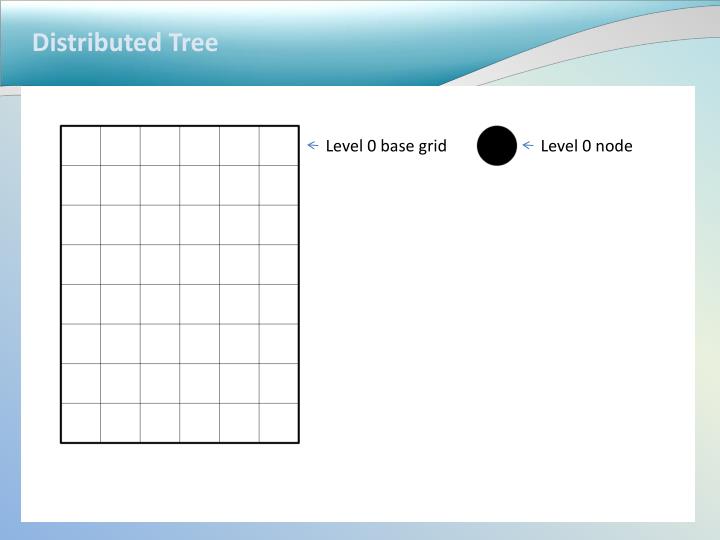The image features a detailed diagram set against a layered background. At the top, there's a blue banner with the title "Distributed Tree" written in bold, white, capitalized letters. The top border also includes a light blue and purple gradient design with flowing lines, adding an element of creativity and style.

Below the banner, the image transitions into a grid section. This section includes a white square, inside which sits a black rectangle. Within this black rectangle is an 8x6 grid, comprised of smaller grid lines. 

On the right edge of the image, there are two annotations. The first annotation is a blue arrow pointing left, labeled "Level 0 Base Grid" in black text, directing attention to the grid. The second annotation features a filled black circle with a blue arrow pointing left, marked "Level 0 Node," indicating a specific spot on the grid. The combination of structural elements and annotations gives the impression that this might be a part of a complex diagram, possibly related to a game or an information grid.